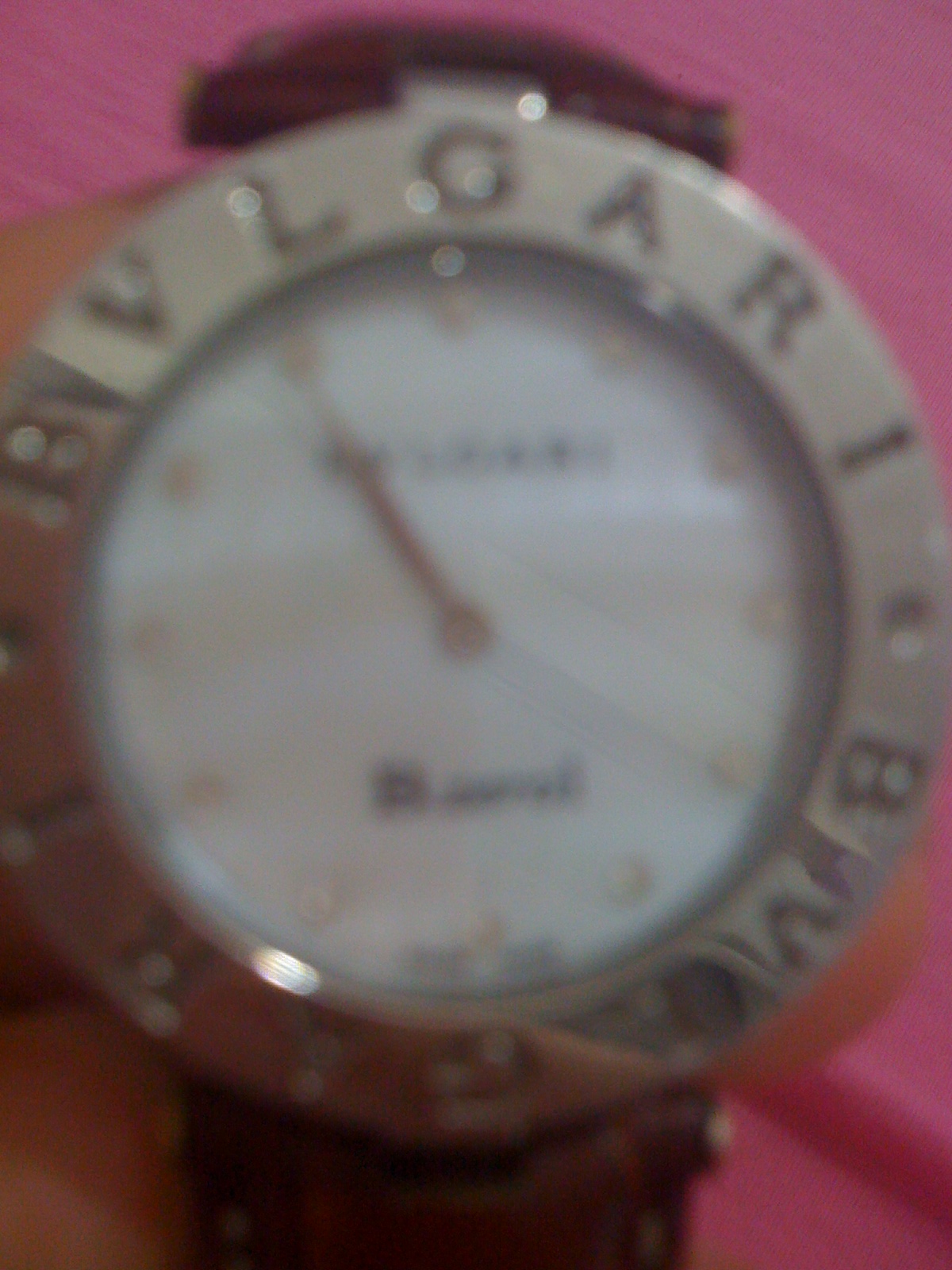A blurred image depicts the face of a Bulgari wristwatch, set against a backdrop of rich red fabric. The white dial prominently features the brand name "BVLGARI" engraved in black text along the top curve, with the letters B-U-L-G-A-R-I spaced intricately around the circumference. The hour hand points towards 11 o'clock, while the black minute hand adds contrast against the white background.

Dark, meticulously arranged dots serve as hour markers along the outer edge of the watch face. A faint light reflection distorts the clarity of the glass or plastic covering the dial, casting an ethereal glow on the inner side of the frame. The watch case, predominantly silver, gleams subtly in the ambient light, complementing the black text and providing an elegant border to the timepiece. Black text is also present at the bottom curve of the dial, adding to the detailed design. Silver wrist straps extend from the top and bottom of the watch case, hinting at the sophisticated design and craftsmanship synonymous with Bulgari watches.